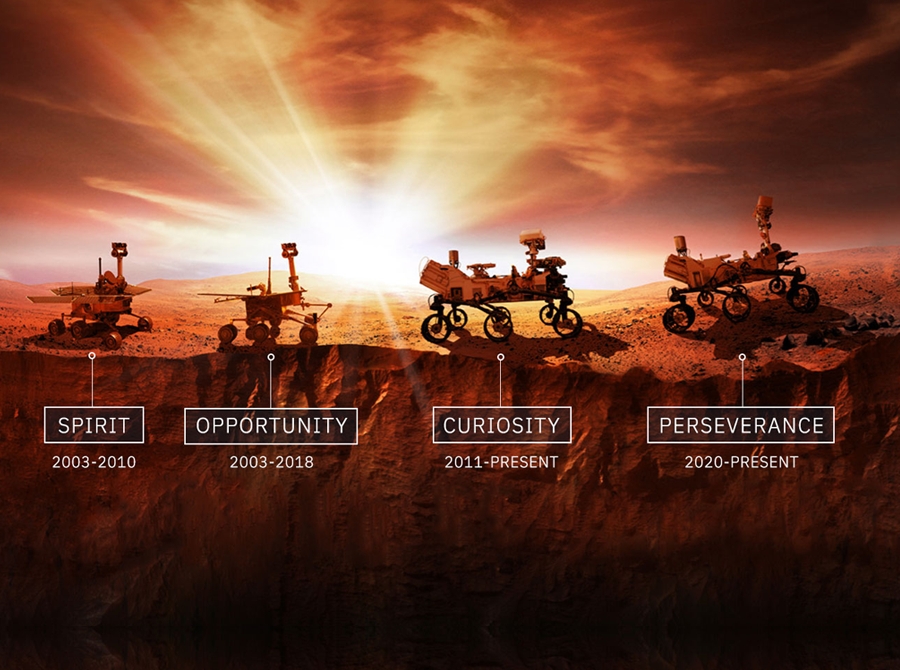This diagram is a detailed digital illustration showcasing the four Mars rovers on the Martian surface, ordered from left to right: Spirit, Opportunity, Curiosity, and Perseverance. Each rover is depicted in profile, seemingly driving from left to right across a rocky Martian landscape under a reddish dark sky with the sun rising over the horizon. 

Spirit and Opportunity, both operational from 2003, are similar in size with six smaller wheels and a camera mounted on top. Spirit's mission lasted until 2010, while Opportunity continued until 2018. In contrast, Curiosity and Perseverance, active from 2011 and 2020 respectively, are larger with six spoked wheels and more substantial bodies featuring multiple cameras. Curiosity and Perseverance are about the same size, significantly longer and more robust compared to the earlier rovers.

Each rover is labeled with a call-out leader to a rectangle below, indicating its name and the duration of its mission. The whole scene is set against the craggy, reddish terrain of Mars, capturing the evolution and increasing complexity of these exploratory vehicles.